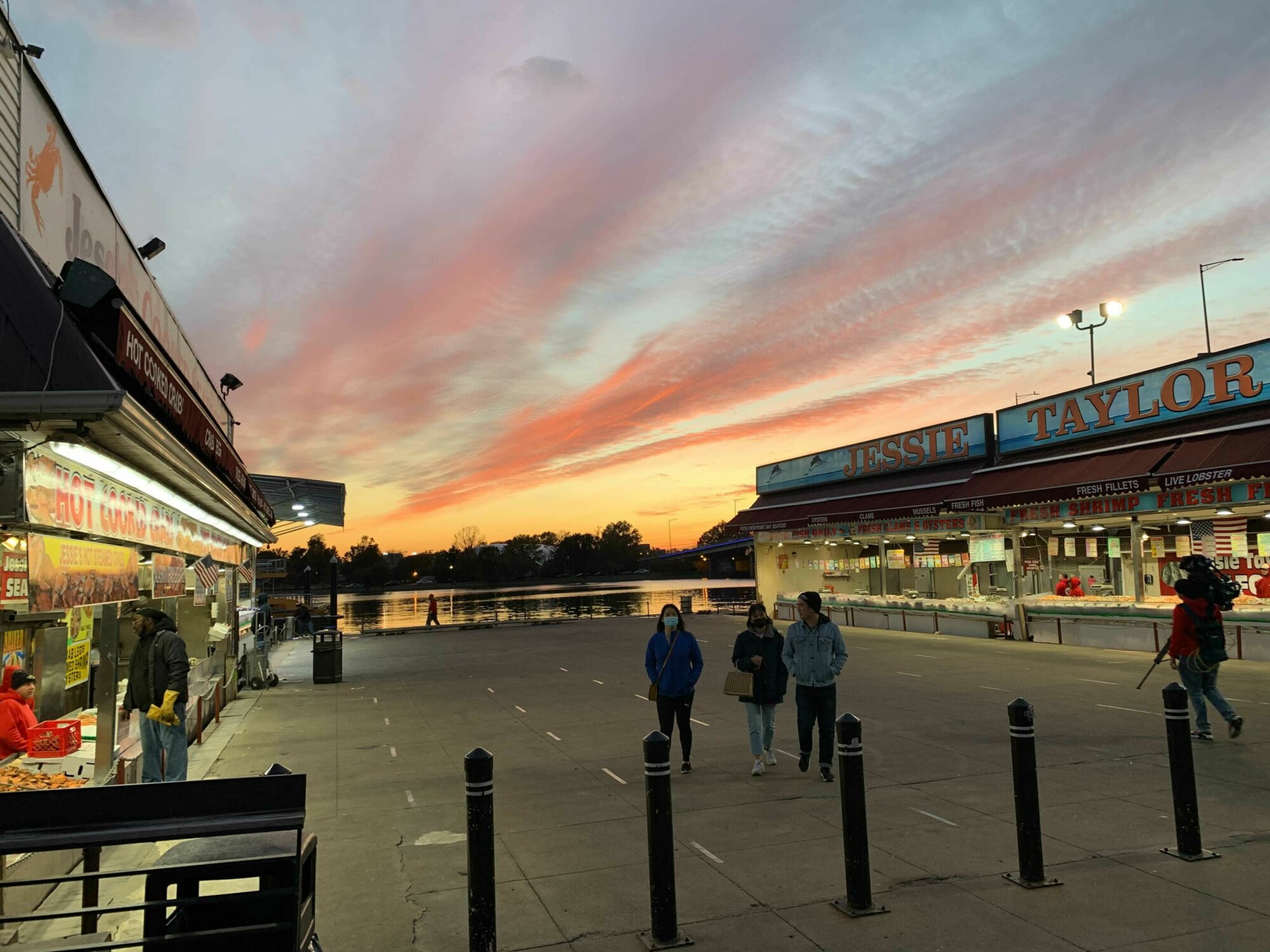The landscape-oriented photograph captures a bustling boardwalk scene set against a stunning sunset. On the right-hand side, a row of food stalls is visible, with a prominent sign reading "Jesse Taylor" in red font on a blue background. The left-hand side also features vendors, one of which sells hot chocolate. The shops are still open, their windows glowing with light. The boardwalk itself is dark gray and busy with activity. In the center of the image, three individuals walk together: one dressed in blue, another in black with blue jeans, and the third in gray with black pants, with one wearing a mask. To the left, a man appears to be ordering food from a stall. The background showcases a serene body of water beside a tree-lined shore, under a sky painted with the wispy hues of a pink, yellow, orange, and blue sunset. The water's surface is dark, no longer reflecting the sun’s rays. In total, five people are captured in this lively and picturesque scene.